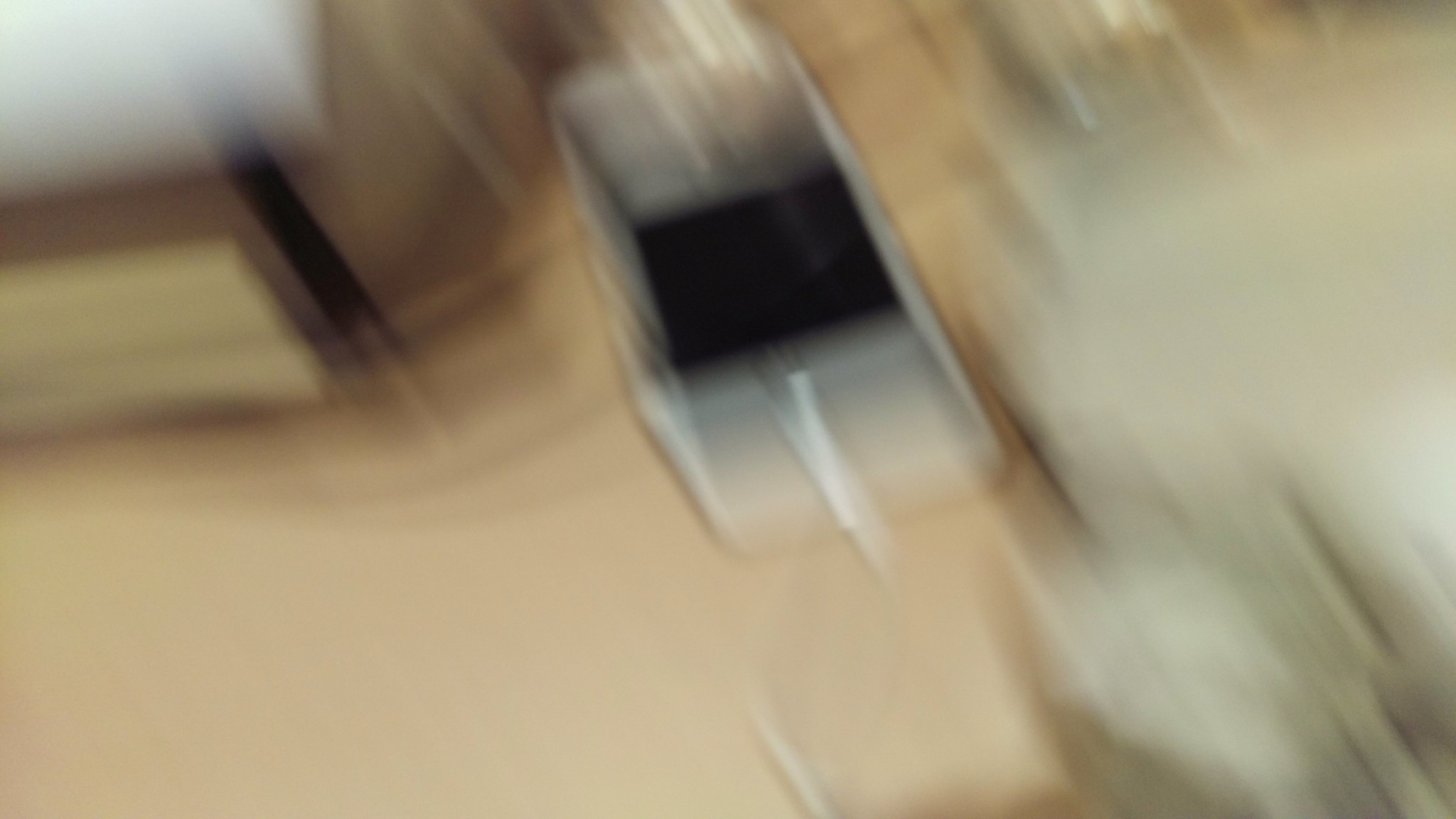This photograph captures an extremely blurry scene of what appears to be a personal desk setting, possibly taken by accident or in motion. The central focus is a brown wooden desk, upon which an older model iPhone, connected to a white charging cable, is positioned. To the left of the phone, there are indistinct fragments that could be parts of a computer or a base, though the blurriness makes it difficult to be certain. The right side of the image is equally hard to decipher, but it shows additional items spread across the wooden surface. The overall impression is of a cluttered desk space caught in a moment of motion or by inadvertent capture.